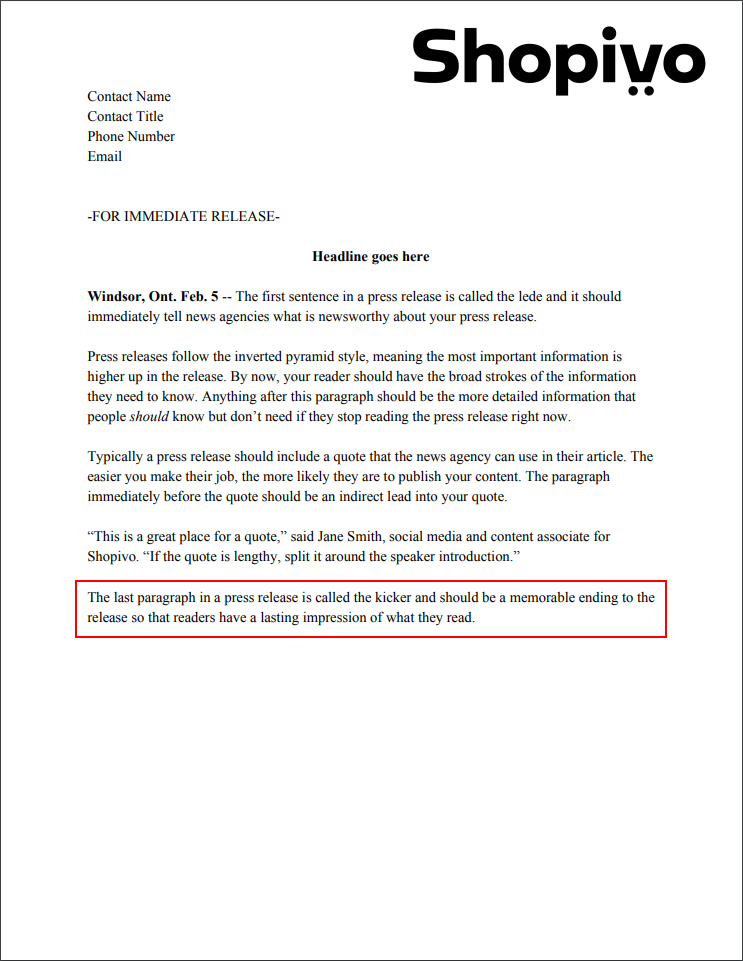This image features a scanned template of a press release letter under the letterhead "ShopiVu." At the top-right of the page, "ShopiVu" is prominently displayed in black text. On the top-left, several bullet points list contact information fields: contact name, contact title, phone number, and email address. Directly below is the phrase "FOR IMMEDIATE RELEASE" followed by a placeholder text "Headline Goes Here" and an indication that the template originates from Windsor, Ontario, dated February 5th.

The body of the template explains key components of a press release format. It starts by defining the "lede" or lead as the initial sentence that should immediately convey the newsworthiness to news agencies. The structure of the press release follows the inverted pyramid style, placing the most critical information at the beginning, ensuring readers grasp essential points quickly.

Subsequent paragraphs provide more detailed information that becomes increasingly specific, with the understanding that readers may opt out after the primary details. The template recommends including a quote from a relevant authority to facilitate media usage, exemplified by a line for a quote attributed to "Jane Smith, Social Media and Content Associate for ShopiVu." The final section, highlighted with a red rectangle, is designated for the "kicker" paragraph, intended to leave a memorable impression on the reader.